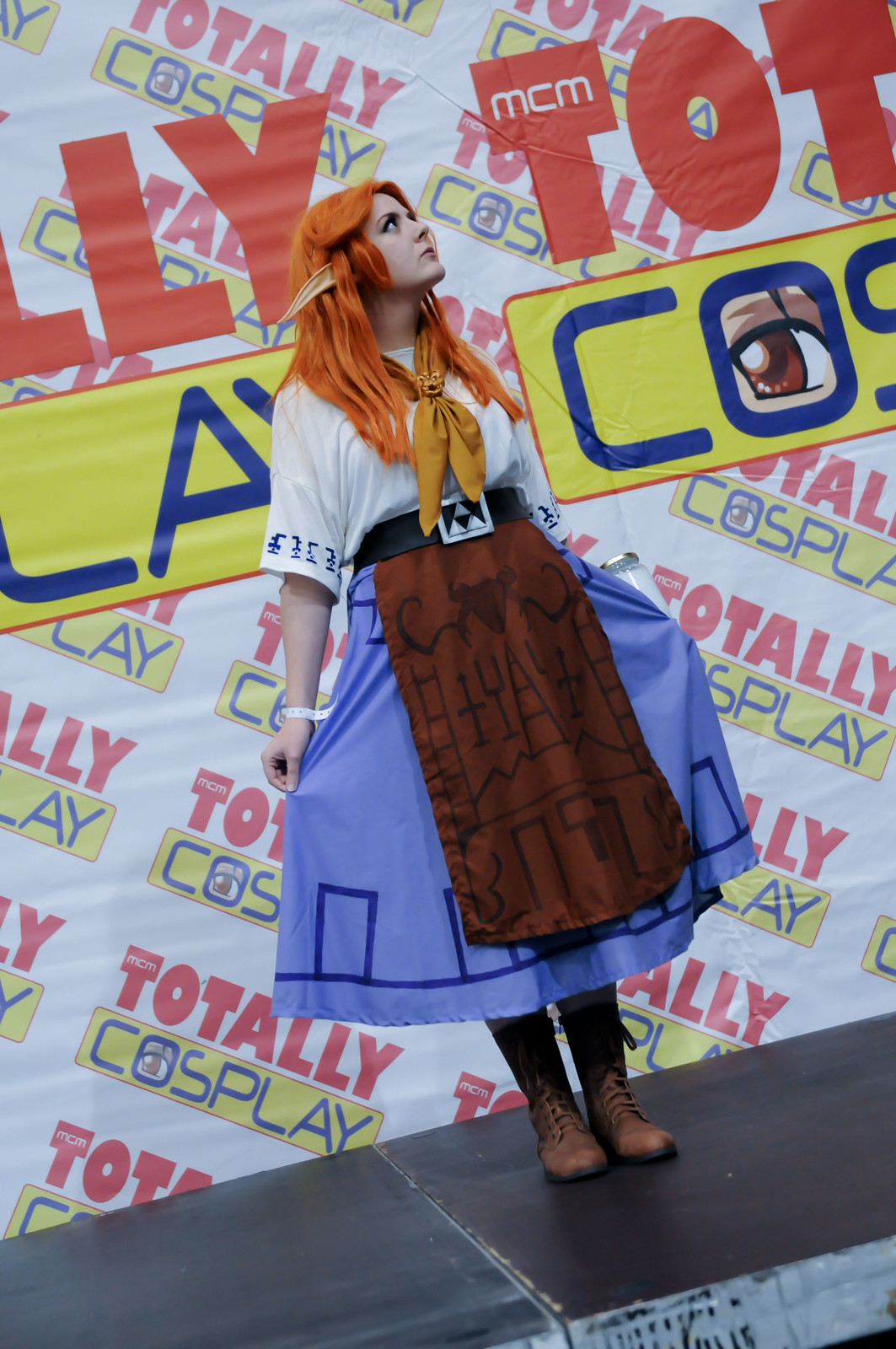The image captures a woman cosplaying a character, likely from The Legend of Zelda series, on stage at a cosplay event. The stage backdrop prominently features the words "TOTALLY COSPLAY" in all caps, with "TOTALLY" in red and "COSPLAY" in yellow. The cosplayer herself is wearing an elaborate costume: she has long, mostly orange hair and pointed elf ears, indicative of a fantasy character. Her outfit comprises a white short-sleeve shirt adorned with Asian script, an orange scarf across her chest, and a blue skirt with dark blue lines. Over her skirt, she wears a dark brown apron. Her waist is cinched by a thick black belt decorated with three triangles forming a Triforce symbol. She also wears brown leather boots with laces. The woman is posed with her face turned toward the top right corner of the image, both hands holding out the fabric of her skirt, and her feet are pointed toward the bottom right. The image is taken from a slight angle that captures her standing on a black stage with a gray side background, adding depth to the scene.